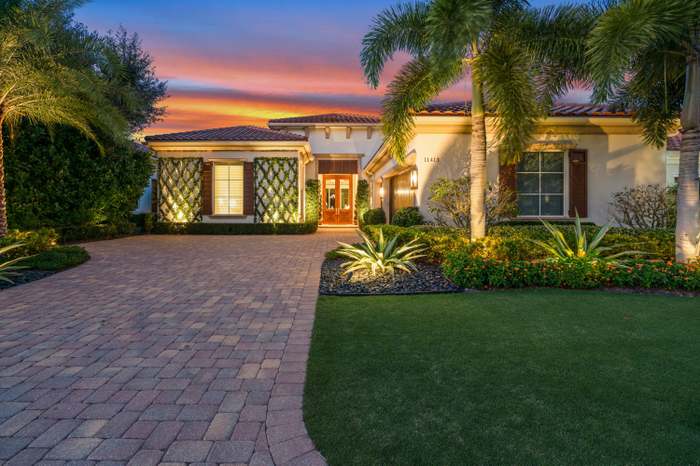The image captures a single-story, Spanish-style home during a vibrant sunset. The sky displays an array of hues—blue, pink, orange, and yellow—creating a dramatic backdrop. In the foreground, a meticulously laid brick driveway leads up to the home, flanked by a beautifully manicured, lush green lawn on the left side. The exterior of the house appears to be a canary yellow or beige color complemented by a red-tile roof. 

The front of the house features a striking red door with two glass windows, framed by an awning above. On either side of the door, there are identical six-pane windows, one of which has a lattice design. Both windows are illuminated from the inside, adding warmth to the scene. The house is adorned with palm trees and other tropical plants in a thoughtfully sectioned landscape, indicating a tropical location, perhaps Florida.

Security and night lighting around the building give it a well-maintained and safe appearance. The overall scene is one of serene elegance, accentuated by the soft, fading light of dusk.